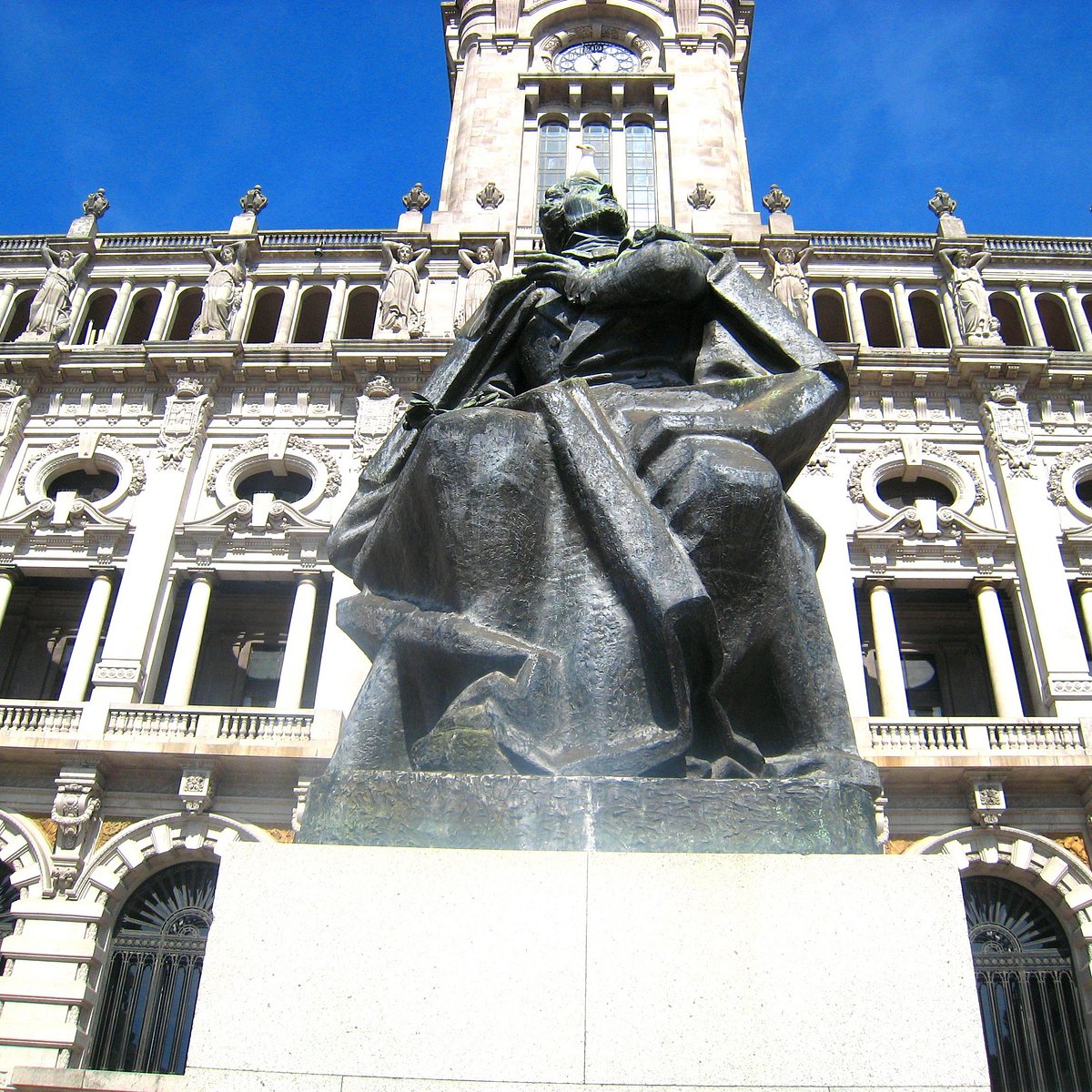The photograph captures a striking statue of a man, possibly from the Napoleonic era, seated on a large, square plinth and draped in a coat that envelops him like a blanket. The man, adorned with a beard and a cape, gazes upwards over his left shoulder, his hand placed on his chest. This statue is positioned prominently in front of an opulent Renaissance-style building, characterized by its white façade, numerous archways, columns, and an elaborate array of statues along its upper sections. Female statues with their hands behind their heads adorn the building, which also features circular windows and a prominent balcony above the first floor. The building's centerpiece is a clock tower displaying the time at 12:55, flanked by bright blue sky. The base-level windows are secured with metal cages, hinting it might be a significant political or government structure. The setting appears to be a public square, commonly found in European cities.